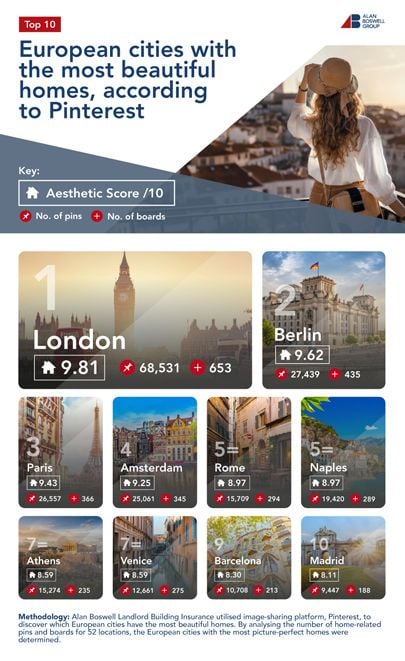Website for Allen Booking Group displaying curated travel destinations worldwide. At the top of the page, a captivating image of a woman gazing over an expansive cityscape sets the tone. Positioned next to the image, a header reads: "European Cities with the Most Beautiful Homes, According to Pinterest." Below this title, the website features key metrics for each city, including an aesthetic score, the number of Pinterest pins, and the number of boards.

Ranking the cities:

1. **London**: 
   - Aesthetic Score: 9.81
   - Number of Pins: 68,531
   - Number of Boards: 653
   
2. **Berlin**: 
   - Aesthetic Score: 9.62
   - Number of Pins: 67,439
   - Number of Boards: 435
   
3. **Paris**: 
   - Aesthetic Score: 9.43
   - Number of Pins: 36,557
   - Number of Boards: 366
   
4. **Amsterdam**: 
   - Aesthetic Score: 9.25
   - Number of Pins: 25,061
   - Number of Boards: 345
   
5. **Rome**: 
   - Aesthetic Score: 8.97
   - Number of Pins: 15,709
   - Number of Boards: 294

This ranking highlights Europe's most beautiful cities, according to aesthetic appeal and popularity on Pinterest.